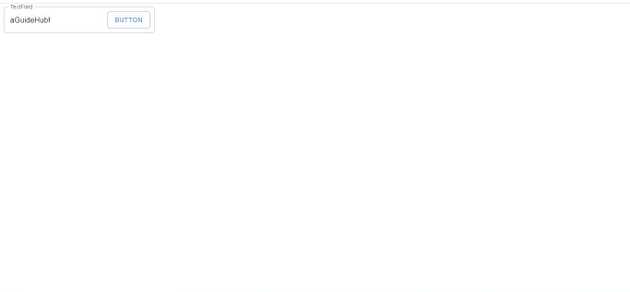The image depicts a predominantly empty page, characterized by a minimalistic design set against a white background. In the top left corner, there is a small icon accompanied by the text "A Guy's Hubby." Additionally, a text button is present nearby. The color palette is restricted to shades of blue and black. Beyond these minimal elements, the page remains devoid of any other content or details.